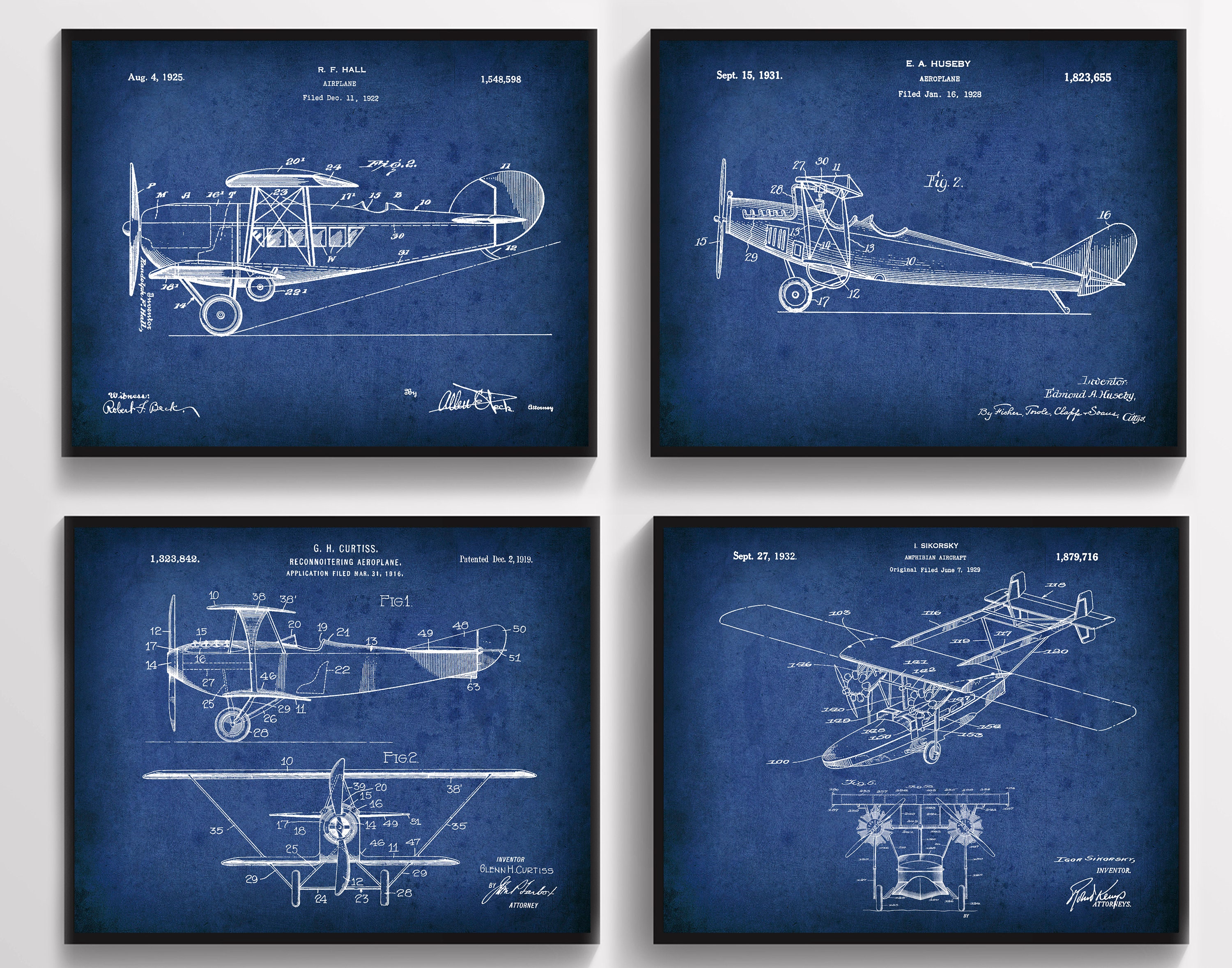The image displays four meticulously drawn blueprints of different airplanes, arranged in a square on a blue background, typical of old architectural blueprints. Each blueprint features white symmetrical drawings of the airplanes and corresponding technical specifications, including dates, names, and patent numbers. 

At the top left, the first blueprint dated August 4th, 1925, showcases the RF Hall Airplane with a side profile drawing of the aircraft. Adjacent to it on the right, the second blueprint, dated September 15th, 1931, depicts the EA Hughes Bee Airplane with the wings removed, revealing internal structure details. Below, on the left, the third blueprint, dated December 2nd, 1919, features the G.H. Curtis Reconditoring Aeroplane, illustrating both a front view and a side view of the airplane. The fourth blueprint, located to the right and dated September 27th, 1932, shows the L. Sikorsky Amphibian Aircraft with a diagonal top view and a front view.

Each blueprint includes detailed but somewhat illegible text, numbers indicating patent identifiers (e.g., 1,548,592; 1,823,655; 1,823,842; 1,879,716), and signatures at the bottom. The unified blue and white color scheme amplifies the historical and technical essence of the blueprints, all encased within a prominent black border that outlines the entire image.